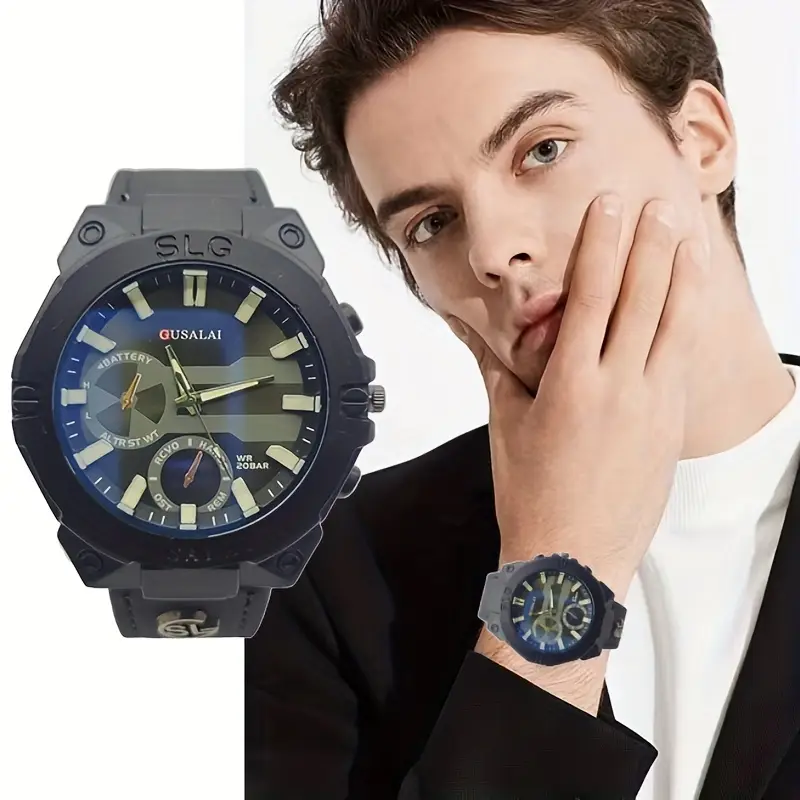In this advertisement for the Gusolani watch, the composition showcases both an extreme close-up of the timepiece on the left and a young male model on the right. The watch face, featuring a circular design with a gray frame and a protective glass cover, displays Roman numerals and an intricate background with an atomic symbol beneath the hands. The time reads approximately 11:12. The watch has a black band with hour notches and the brand name "Gusolani" elegantly displayed.

The model, a young man with short to medium-length brown hair, cradles his chin with his right hand, prominently displaying the watch on his wrist. He is dressed in a black jacket layered over a white t-shirt. The color palette in the advertisement includes black, white, dark blue, a hint of red, gray, and brown tones. The photo's setting remains ambiguous, leaving it unclear whether it was taken indoors or outdoors, or during day or night time. The model slightly tilts his head, further emphasizing the sophisticated design of the watch.